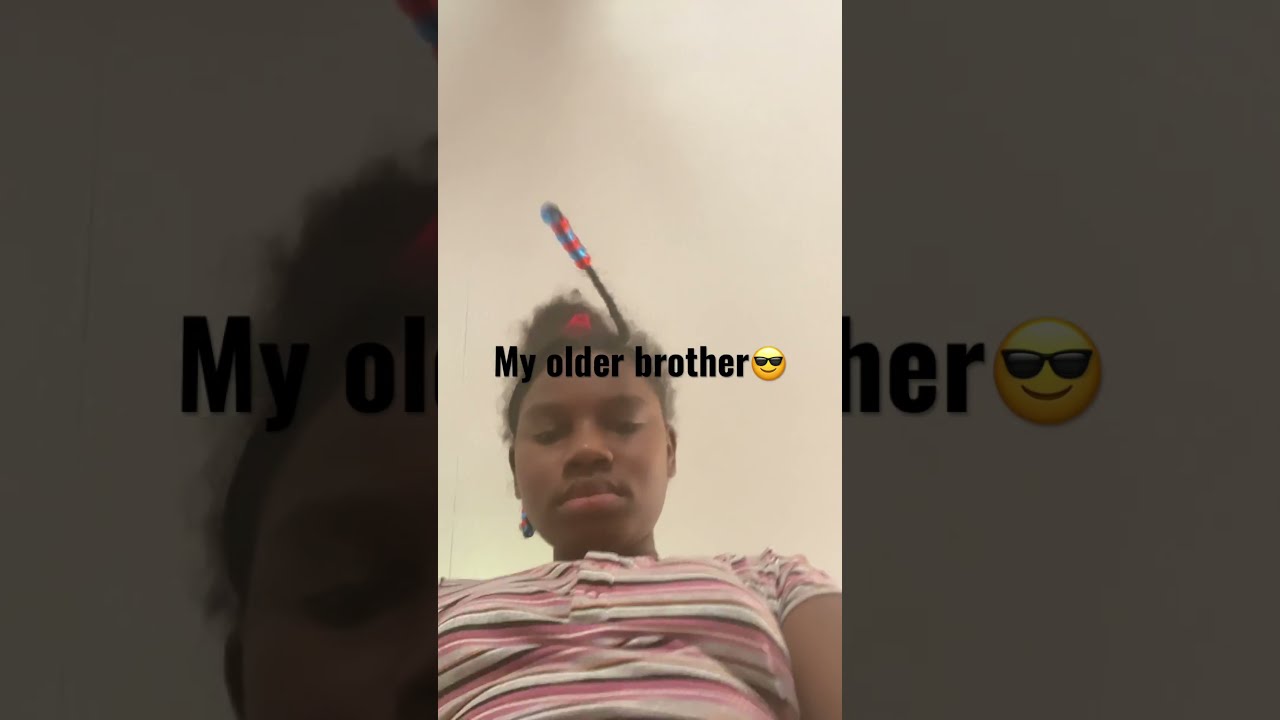The image is a screenshot of a portrait video and is divided into three sections. The center section features a black girl with her hair styled in a bun, and a braid adorned with red and blue beads sticking out like an antenna. She is wearing a tight-fitting shirt with white, pink, and maroon stripes. The background is a plain white-beige ceiling. She gazes downward at the camera held low, capturing her from the belly up. 

Text overlays the middle section, reading "my older brother" in a black sans-serif font, accompanied by a sunglasses emoji. The girl's face is expressionless, and the context implies some innuendo or a humorous TikTok post. 

The left and right sections are darkened, zoomed-in portions of the central image. The left shows just her upper face, and the right focuses on the sunglasses emoji beside the text. This creates an enlarged backdrop framing the central portrait.